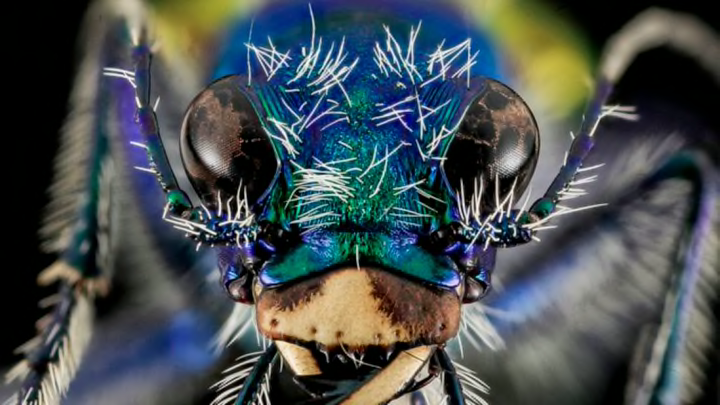This striking close-up macro image captures the detailed and vibrant face of a fly with remarkable clarity. The fly's head dominates the composition, showcasing its vivid colors that range from royal blue and electric turquoise to hints of bright green. The intricate surface is adorned with flicks of white hairs, acting as sensors, that create a textured and almost furry appearance. The fly's large, shiny brown eyes are positioned on either side of its face, reflecting light and providing a stark contrast to its colorful head.

Central to the image is the fly's nose, which is illuminated in such a way that it appears to shimmer in gold tones, though it likely consists of more natural brown and beige hues. Below the nose, the mouth area transitions into a tan and brown region with tan-colored mandibles extending downward.

Protruding from the sides of the head are long legs, also featuring electric blue and white spiked hairs, which extend slightly beyond the frame. The partially visible antennae add to the sense of intricate detailing with their white hairs. The background remains blurry, ensuring that every focus remains on the fly’s mesmerizing and vibrant face, capturing the complex textures and vivid colors that make this close-up image exceptionally detailed and captivating.